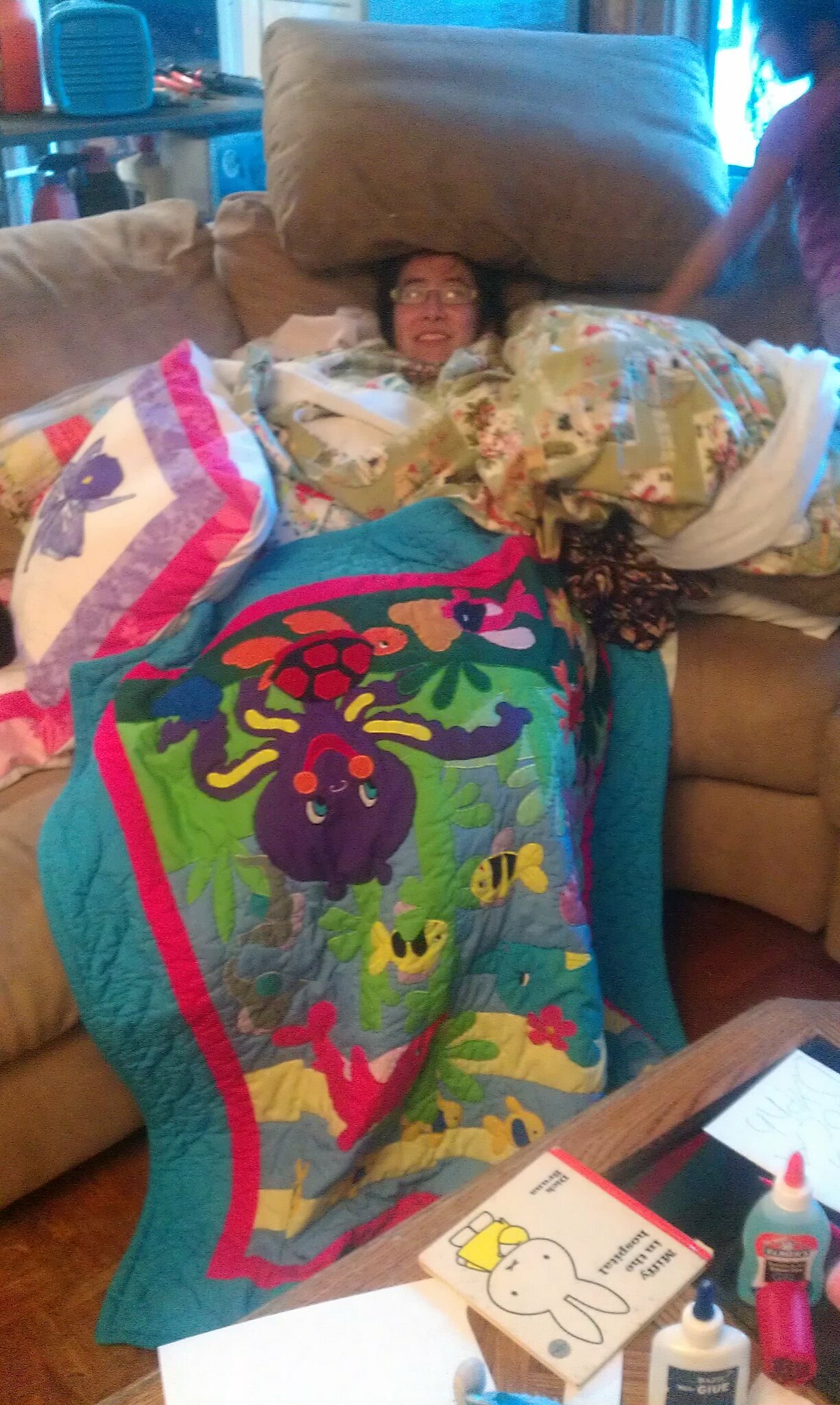In the cozy corner of a beige sectional couch, a person sits nearly enveloped by a collection of colorful pillows and blankets. With dark hair and glasses, they smile, their head the only part visible amidst the array of cushions. Resting on their legs is a quilted blanket featuring an underwater design with a large purple octopus, yellow and black fish, green marine plants, a blue dolphin, and an orange-pink turtle, although the blanket appears to be upside down. Flanking the person are various pillows: on the left, a white pillow adorned with purple and pink borders and a central purple flower, and a green printed pillow on the right. In the bottom right corner, a coffee table holds several glue sticks, scattered pieces of paper, and a small book with a bunny on the cover. Adding to the lively scene, a little girl in a purple shirt is partially visible, her arm in motion as she seems to be jumping on the couch.